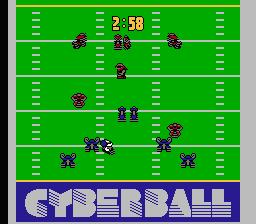This image is a detailed screenshot from the NES video game "Cyberball," a futuristic take on football. The field is depicted with bright green turf, divided by multiple horizontal lines, with white lines marking every ten yards and yellow lines at the bottom and back. The top of the image features a timer set at 2 minutes and 58 seconds, displayed in light orange. Players on the field are color-coded, with some wearing blue and others in red. At the bottom of the image, there's a blue rectangular banner with the word "Cyberball" written in grayish-white text. The sides of the image have gray and black borders, contributing to the overall retro aesthetic. The screenshot captures the essence of the early sci-fi sports game, blending traditional football elements with a futuristic twist.